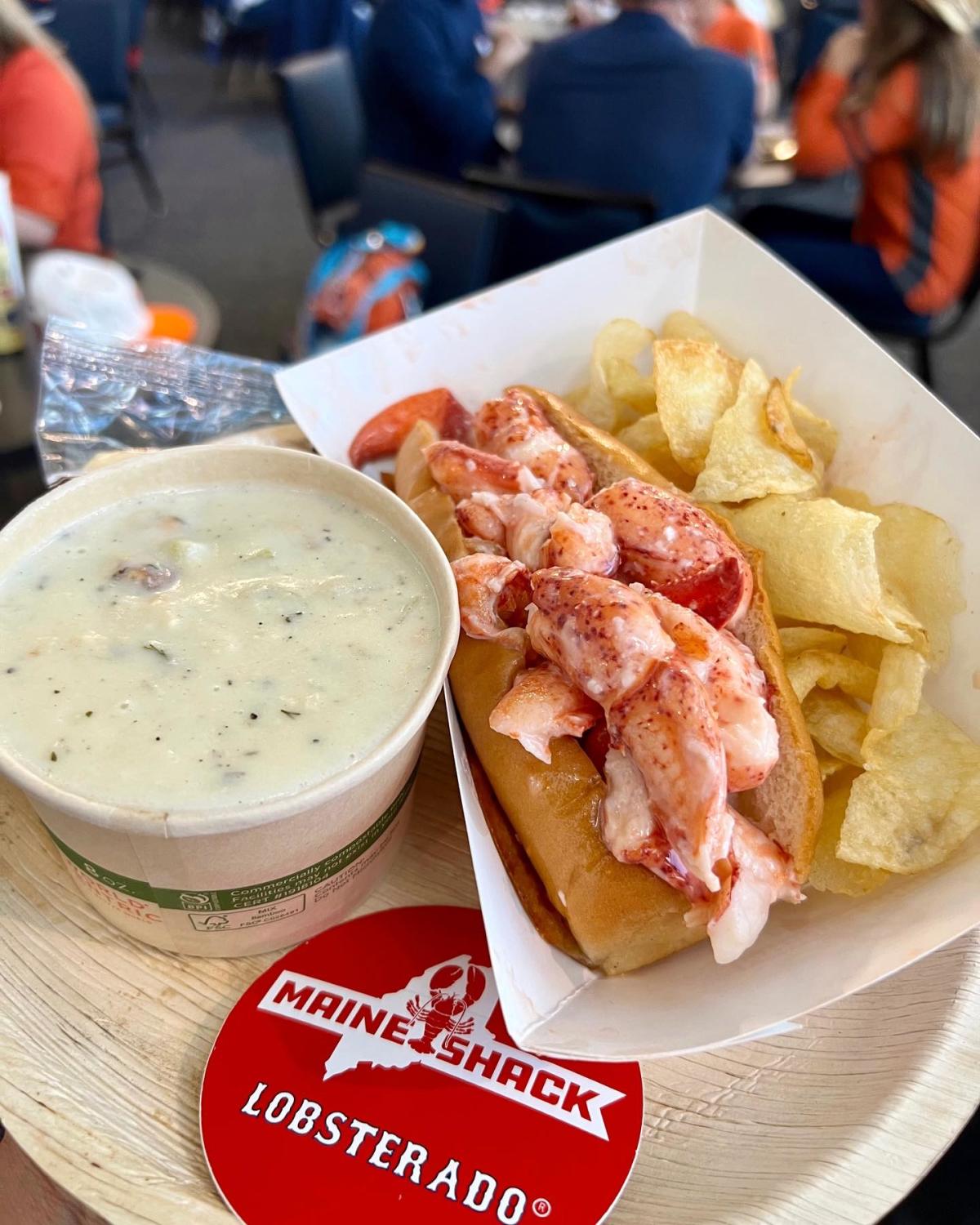This image captures a close-up of a savory meal at a restaurant called Main Shack Lobsterado. Centered on a paper plate with a wood-like pattern, the star of the meal is a delectable lobster roll nestled inside a small paper takeout container, accompanied by a portion of crispy potato chips. To the side sits a small styrofoam cup wrapped in a green band, containing a creamy clam chowder, garnished with herbs and seasonings. Adding a touch of branding, a small round red sign on the plate reads "Main Shack Lobsterado" with a lobster illustration. In the blurry background, other diners can be seen at their tables, creating a bustling restaurant atmosphere. A plastic bag with to-go cutlery peeks out from behind the chowder, completing the dining setup.